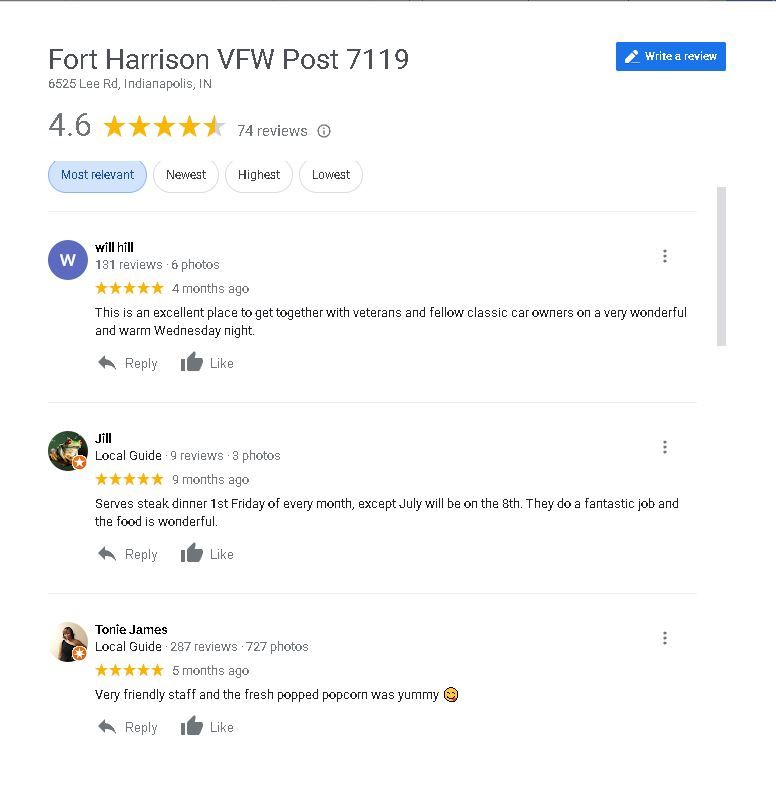The image showcases a review page for Fort Harrison VFW Post 7119. The address 6625 Lee Road, Indianapolis, Indiana, is prominently displayed below the header. In the top right corner, against a blue background, there's an option to "Write a Review." The page indicates an overall rating of 4.6 stars based on 74 reviews. Four sorting options are available: Most Relevant (highlighted in blue), Newest, Highest, and Lowest.

Below these options are three detailed reviews. 

1. The first review is by Will Hill, who has a profile icon featuring a "W". Will has contributed 131 reviews and 6 photos. He rates the post 5 stars and shared his thoughts 4 months ago: "This is an excellent place to get together with veterans and fellow classic car owners on a very wonderful and warm Wednesday night."

2. The second review is by a user named Jill, identified as a Local Guide. Her profile icon is a picture of a frog. Jill has posted 9 reviews and 3 photos. She rates the post 5 stars and commented 9 months ago: "Serves steak dinner first Friday of every month except July will be on the 8th. They do a fantastic job and the food is wonderful."

3. The final review featured is by Tony James, also a Local Guide. Tony's profile icon is a picture of a woman, and he has contributed 287 reviews and 727 photos. He rates the post 5 stars and shared his thoughts 5 months ago: "Very friendly staff and the fresh popped popcorn was yummy 😊."

This detailed caption captures each element of the review page in a structured and comprehensive manner.